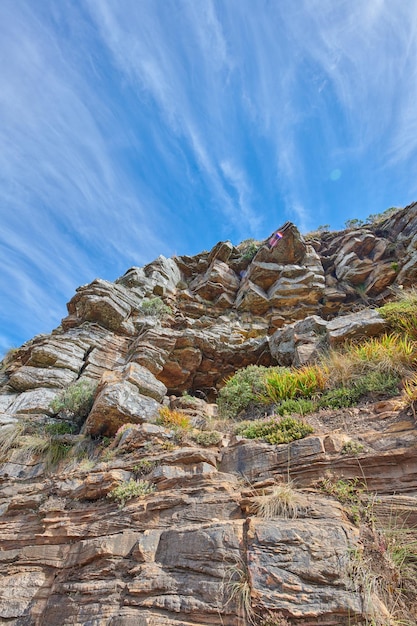The image captures a striking rock formation, photographed from its base with the camera angled upward, emphasizing the dramatic rise of the jagged, sedimentary cliffside. The rocks, composed of various layers of different minerals, reveal a rugged texture adorned with sparse, dry vegetation—mossy patches and small desert shrubs, suggesting an arid landscape with infrequent rainfall. The sky overhead is a brilliant blue with wisps of white clouds, indicative of a bright sunny day, likely around midday. Midway up the formation, a cave-like entrance punctuates the rocky surface. On the middle-right of the image, atop a particularly pointy rock, a flag in pink, blue, white, and red adds a splash of color to the natural scene, standing as a testament to human presence or achievement in this stark, desert environment.